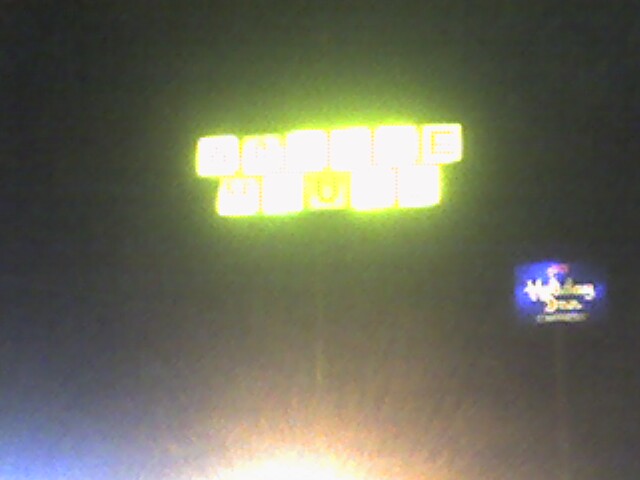This is a nighttime photograph featuring two prominent signs against a pitch-black sky. The central focus of the image is a brightly lit Waffle House sign, characterized by six yellow squares on the top row and five yellow squares on the bottom row. The sign is so intensely backlit that it mostly appears blown out, making it difficult to discern the letters except for a capital 'E' at the end of "Waffle." The metal pole holding the sign is only faintly visible against the dark sky. Below the Waffle House sign, there is a bright white spot of light that casts a glow with an orange and hazy yellow aura. 

To the right of the main sign, there is a Holiday Inn Express billboard. This sign is smaller and features white cursive letters for "Holiday Inn" on a blue rectangular background, and beneath it, the word "Express" in a standard white font. The Holiday Inn sign sits on top of a large post, and although it's slightly less bright compared to the Waffle House sign, it still stands out prominently in the image. The photo is grainy, suggesting it might have been taken with an older camera or digitalized from a non-digital source. The colors appear a bit off, with light leaks creating greenish and blueish hues around the bright areas in the lower corner. The overall image is quite striking due to its intense contrasts and the overwhelming brightness of the signs set against the inky night sky.